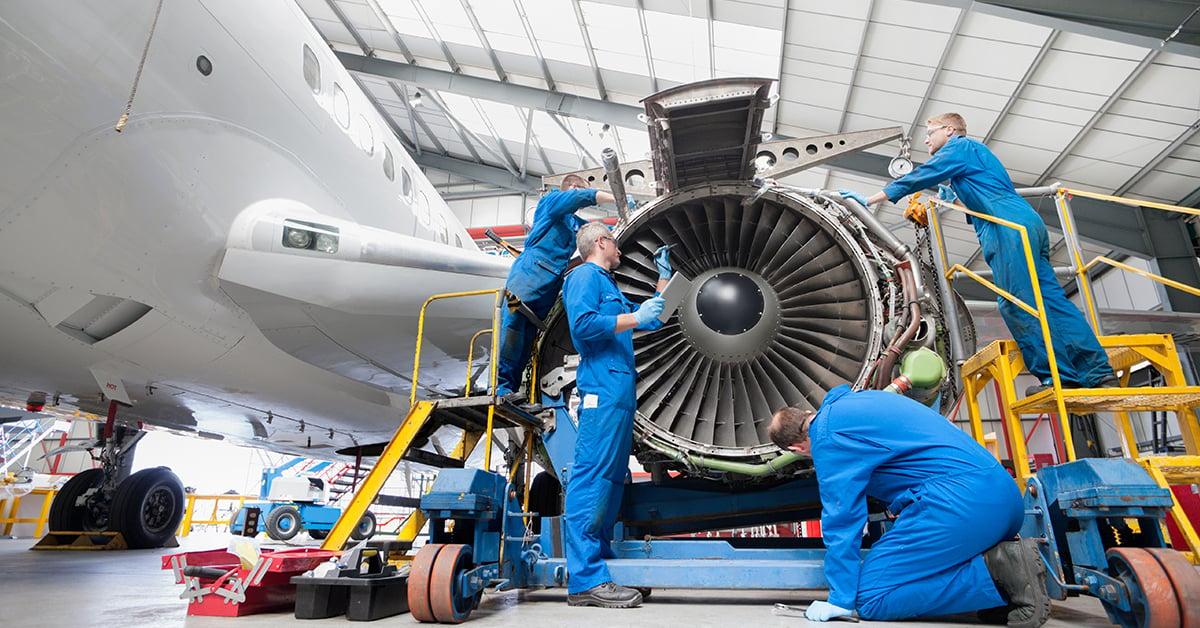In this detailed color photograph, four male airplane mechanics, donned in blue jumpsuits and gloves, are diligently working on a white aircraft engine within a pristine, brightly lit hangar. The mechanics are positioned around the engine: two are standing on yellow stairways to access the upper parts, while the other two are stationed on the ground, tending to the front and lower sections. The airplane, devoid of any graphics, showcases its landing gear prominently. Sunlight streams through the hangar, illuminating the scene and adding to the clean, organized appearance. The focus of the photo is slightly off-center, enhancing the dynamic composition of the workers and the machinery.